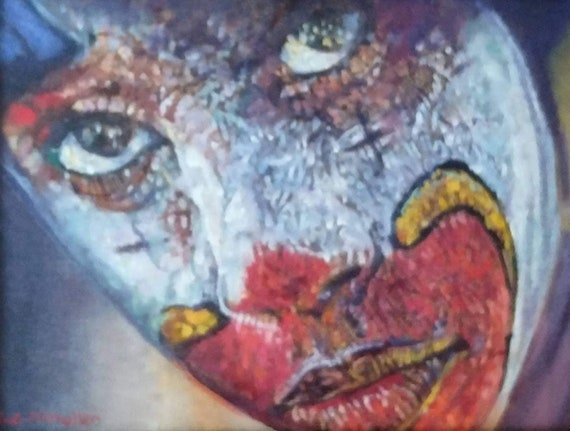This landscape-oriented image is an up-close, slightly blurry photograph of a painting depicting a young boy dressed as a clown. The boy's face is predominantly painted white with large red and yellow accents, giving it a traditional clown appearance. His expression is notably sad, his eyes staring straight ahead, but the color of the eyes isn't clearly visible. The child's forehead has a smear of blue paint, while the area around his eyes features a mix of red and brown hues, including two small black crosses under each eye, positioned more on his cheeks. His nose tip is painted red, and his mouth area is accentuated with a large, vibrant red circle edged with yellow. The image includes a barely legible red signature in the bottom left corner, adding to the artistic quality of the piece.